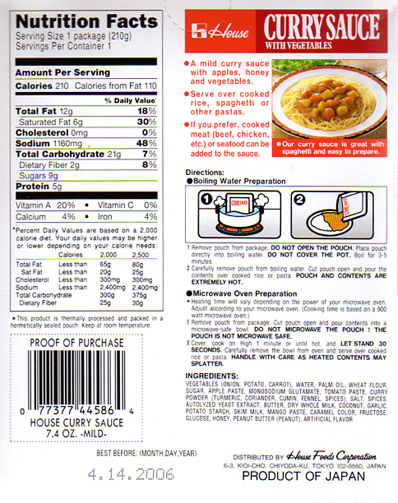This is an image of a label from a product called Curry Sauce with Vegetables. The label describes it as a mild curry sauce flavored with apples, honey, and vegetables, and suggests serving it over cooked rice, spaghetti, or other pastas. The image features an appetizing picture of the dish elegantly presented on a white plate with a red rim. 

The label provides several useful details, including directions for preparation, highlighting options to either microwave or boil the sauce. One side of the label indicates that it is a product of Japan and includes a proof of purchase sticker. Nutritional information is also provided, listing calories, total fat, cholesterol, sodium, protein, and vitamins. Additionally, the label notes the best before date as April 14, 2006, suggesting that the product was bought some time ago.